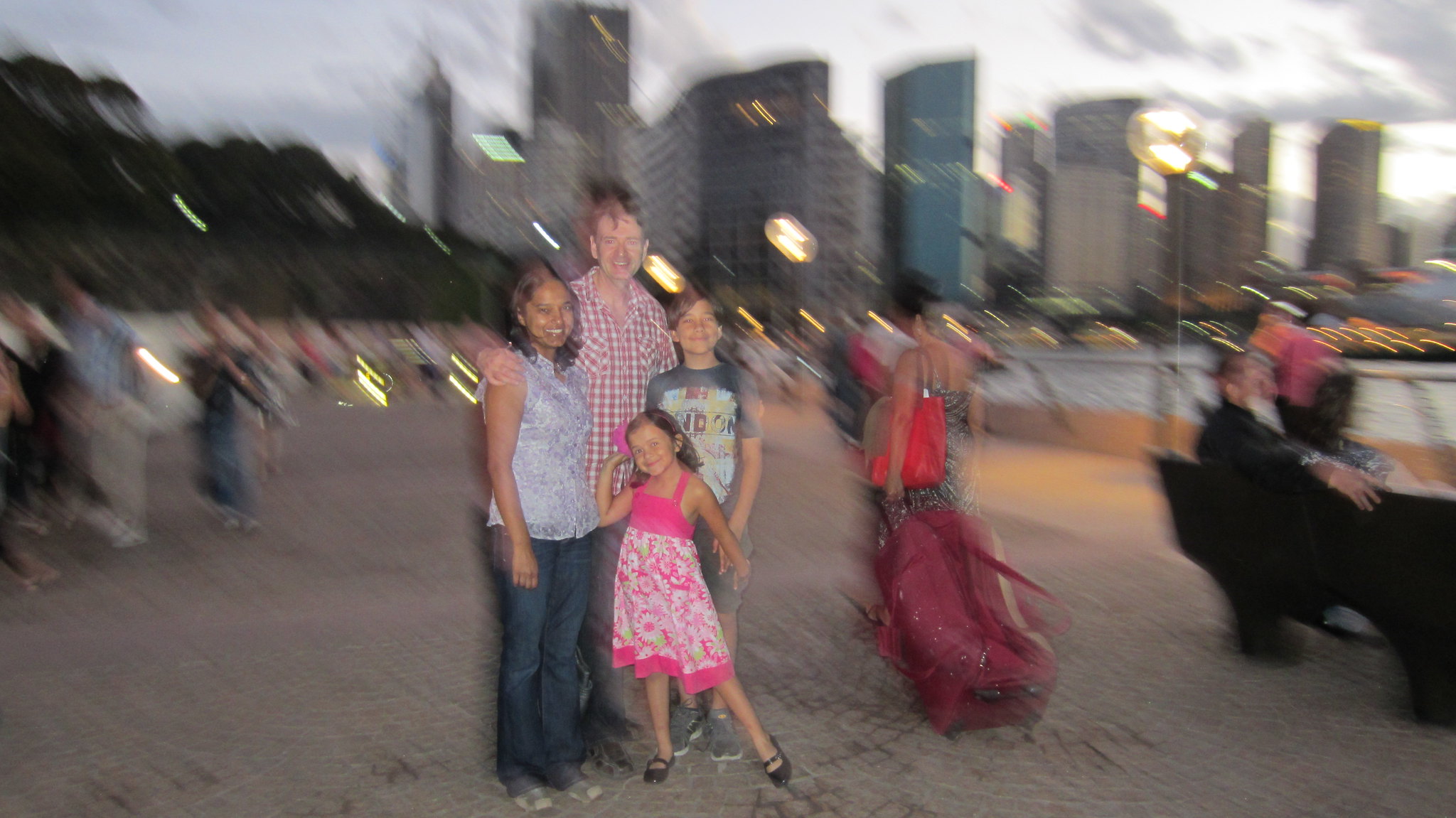A candid real-life photo captures a family of four in what appears to be a coastal or vacation city, possibly Florida or Australia. Positioned on a busy cement walkway bustling with foot traffic, the scene is set either in the evening or on a dark, stormy day, as the lighting is dim. 

The family consists of a white man with short hair wearing a red and white plaid shirt. He stands behind two adults and has his arms around them. On his left is a dark-skinned woman with shoulder-length hair, dressed in a light blue sleeveless blouse and long jeans, with her arms naturally resting at her sides. On his right is a young boy in a t-shirt. In front of the man, centrally located between the woman and the boy, stands a young girl wearing a pink dress adorned with a white floral pattern on the bottom half and dress shoes.

The image is notably blurry, lacking clear focus on the family. The background to the left features dark greenery, while the upper right reveals a cityscape with numerous skyscrapers illuminated by city lights, which appear as streaks due to motion blur, adding to the photograph's dynamic quality.